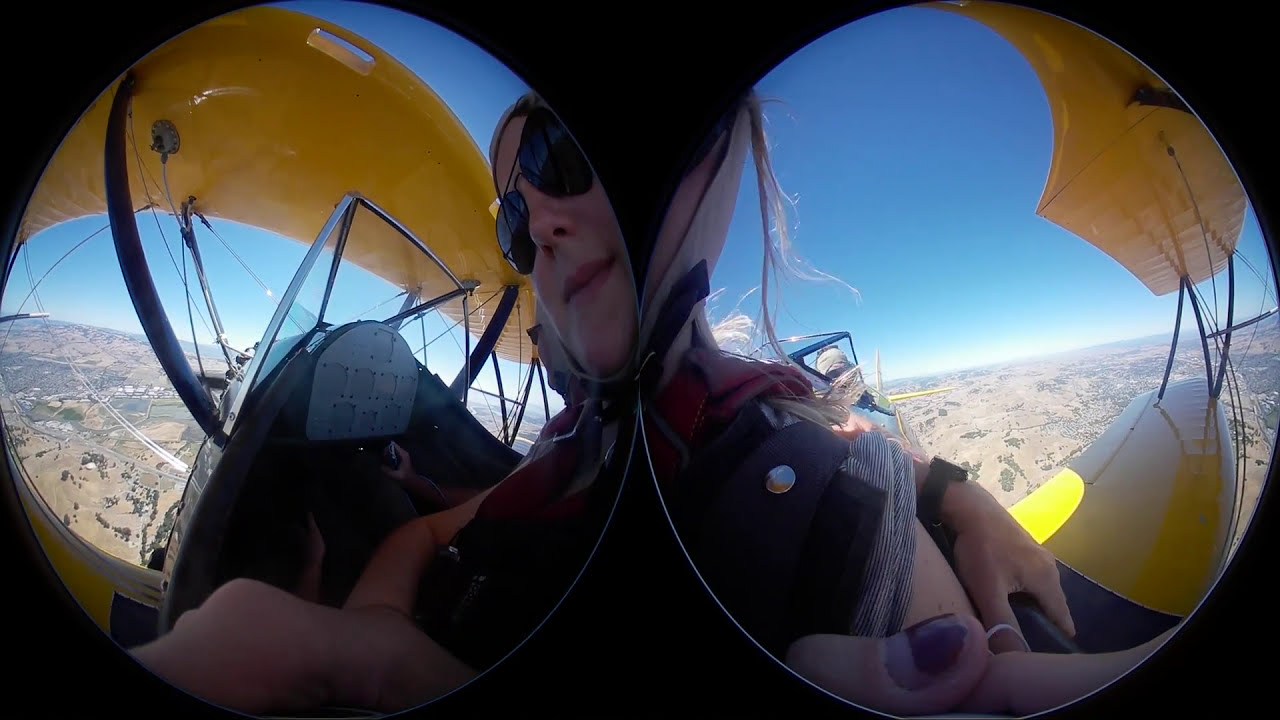In this vibrant photo, taken from the perspective of a passenger in a yellow biplane at high altitude, an exhilarating scene unfolds. The aircraft features an open cockpit, with no enclosing windows or roof, providing an unobstructed view of the clear, sunny skies and the expansive landscape far below. Central to the image is a woman with purple nail polish, seen in binocular perspective. She is wearing sunglasses and some sort of parachuting gear, likely for a potential aerial adventure. The colors in the image are vividly captured, showing hues of black, yellow, blue, tan, pink, red, brown, and gray. The ground beneath, seemingly a vast desert, stretches out into the distance, emphasizing the height and openness of the scene. The overall impression is one of thrill and freedom, with the lady's partially visible face and attire adding a personal, adventurous touch to the composition.